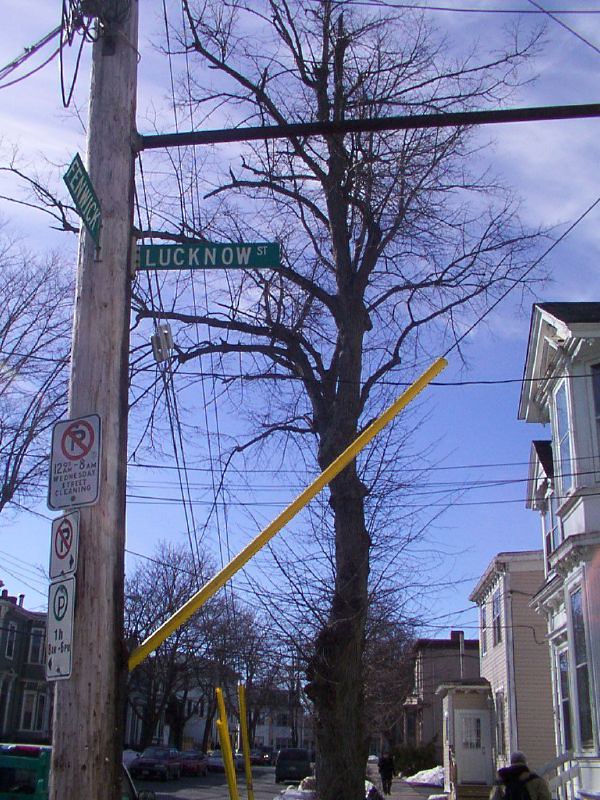The image depicts a weathered telephone pole situated along a residential street. At the very top of the pole, power and communication lines stretch out in various directions. Below, street signs are affixed to the pole; one green sign at the top reads "Lucknow Street," while a slightly bent sign on the left appears to say "Fenwick." Further down the pole, there are three distinct "No Parking" signs. The perspective of the image looks down the sidewalk, flanked by houses on both sides, suggesting a neighborhood that may be on the outskirts of a major city like Chicago or East New York.